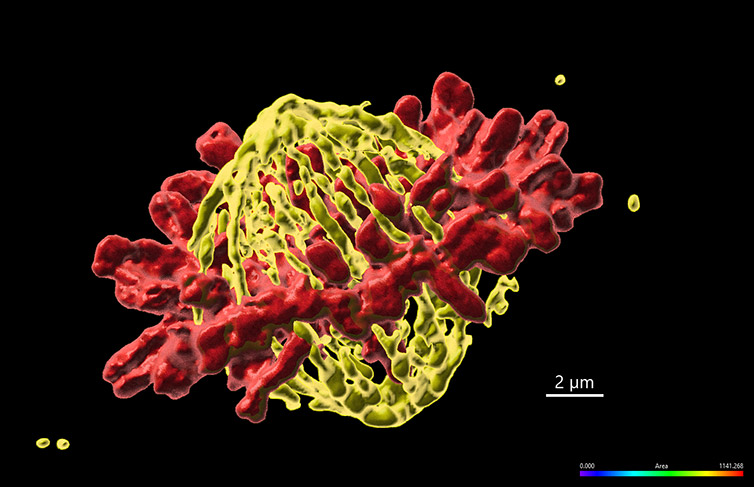This digitally created, animated-looking image is a horizontally-oriented rectangle with a black background. At the center, there is an oval-shaped structure that closely resembles a virus or bacteria. The central body of this structure is yellow with a round surface, and it is enveloped by red protrusions starting from its equator, extending outwards. These red extensions cover the entire middle section of the main body, adding a dynamic, almost spiky appearance. In addition, there are clusters of yellow dots positioned at the upper right and lower left of this central structure. In the lower right corner of the image, "2UM" is inscribed in white, indicating a size reference. Directly below this, a scale bar features a gradient of colors including blue, green, yellow, orange, and red, with white numerical markings denoting specific values. The black backdrop and the vivid colors of the components create a stark contrast, emphasizing the intricate details of the central structure.